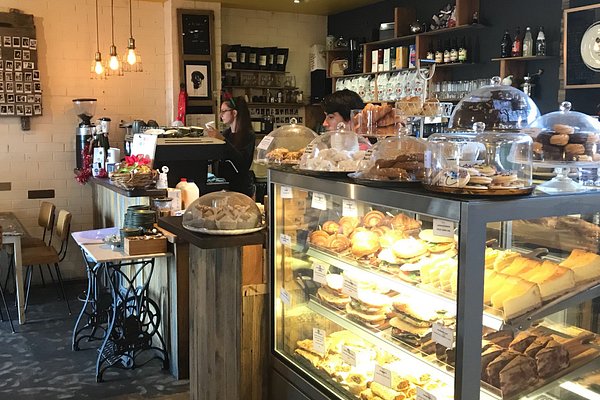In this vibrant and well-lit image of a cozy bakery, the scene is dominated by a prominent glass display case situated in the foreground. This rectangular case showcases three layers of neatly arranged baked goods including bread, cookies, muffins, brownies, cakes, and donuts. The display is internally illuminated, adding a warm, glowing ambiance that accentuates the freshness and appeal of the treats. Atop the case are several glass cake domes, each housing an additional assortment of cookies and pastries, their surfaces reflecting the bright natural light streaming in from outside.

On the counter beside the display case, additional baked items are attractively presented, further enticing customers. To the left of the display case stands a cashier, a lady, assisting a customer, while another worker, a gentleman, moves about behind the counter. This area is backed by a black wall adorned with shelves holding various items, including coffee bean bags and other drink options.

The bakery's welcoming atmosphere is enhanced by a small table with wooden chairs positioned off to the side, inviting patrons to linger and enjoy their purchases. Overhead, stylish hanging lights add to the bakery's charm, completing the picture of a bustling yet inviting culinary destination.